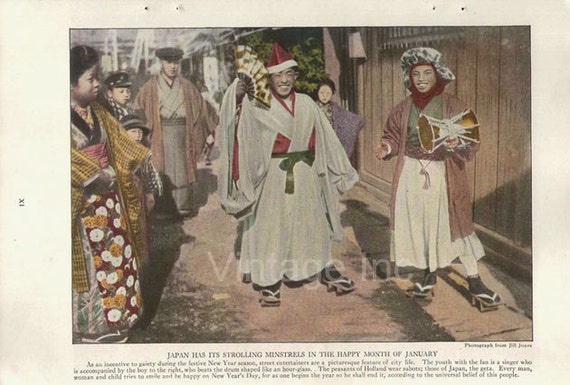This is a vintage color photograph, measuring approximately 4 inches wide by 3 inches high, seemingly clipped from an old newspaper. The image is bordered by a light gray frame, particularly prominent on the top, right, and left sides. At the left side, there is a Roman numeral "IX" in black print. 

The photograph portrays a group of traditional Japanese strolling minstrels, noted as performing in the happy month of January, according to the caption beneath the image. Central to the scene is a man of Japanese descent, smiling at the camera. He is dressed in a long white tunic with a v-neck and a gown, cinched at the waist with a green belt accented by red detailing. His head is adorned with a red hat featuring a white rim and a pointed top, and he holds a traditional fan in his right hand. Sandals with dark gray socks complete his attire.

To his right stands another man, garbed in a dark robe, wearing a distinct black and white hat that caps around the sides of his head. He boasts a red scarf draped around his neck and a green shirt beneath his robe, paired with a white skirt-like bottom. In his left hand, he holds an object, presumably a drum, suggesting his role as a drummer in the minstrel troupe.

On the left side of the central figure is a woman dressed in a traditional kimono (or yukata), contributing to the cultural essence of the scene. Behind them are additional people in traditional dress, watching the minstrels, indicating a moment of cultural celebration or performance.

Across the bottom of the photograph, partially covering the central figure's feet, is a faint watermark reading "vintage ink," further emphasizing the historical and cultural significance of the image.